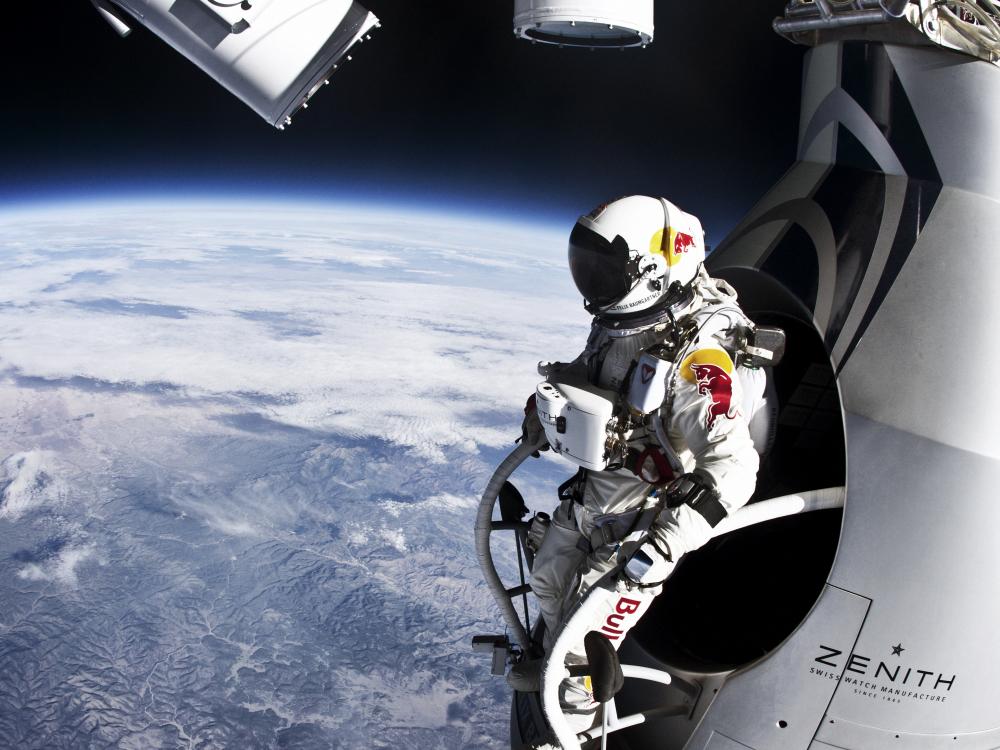This is a highly detailed photograph featuring an astronaut in space, emerging from a circular porthole of a space station or vessel. The backdrop includes the dark expanse of space above, contrasted by the vibrant blues and whites of Earth below, showcasing clouds and mountainous regions. Text on the image reads "Zenith Swiss watch manufacturer," though the date is indistinct. The astronaut, donned in a white suit with black straps and various equipment, has a helmet with a black shield, detailed with a Red Bull logo head-butting a red and yellow circle. Additional Red Bull branding includes an insignia on the left shoulder and the word “BULL” running down the left leg. The astronaut is grasping a white piece of equipment marked "Zenith," which features several small holes, suggesting both branding and functional design. This scene captures the serene yet powerful juxtaposition of advanced technology and the infinite frontier of space.